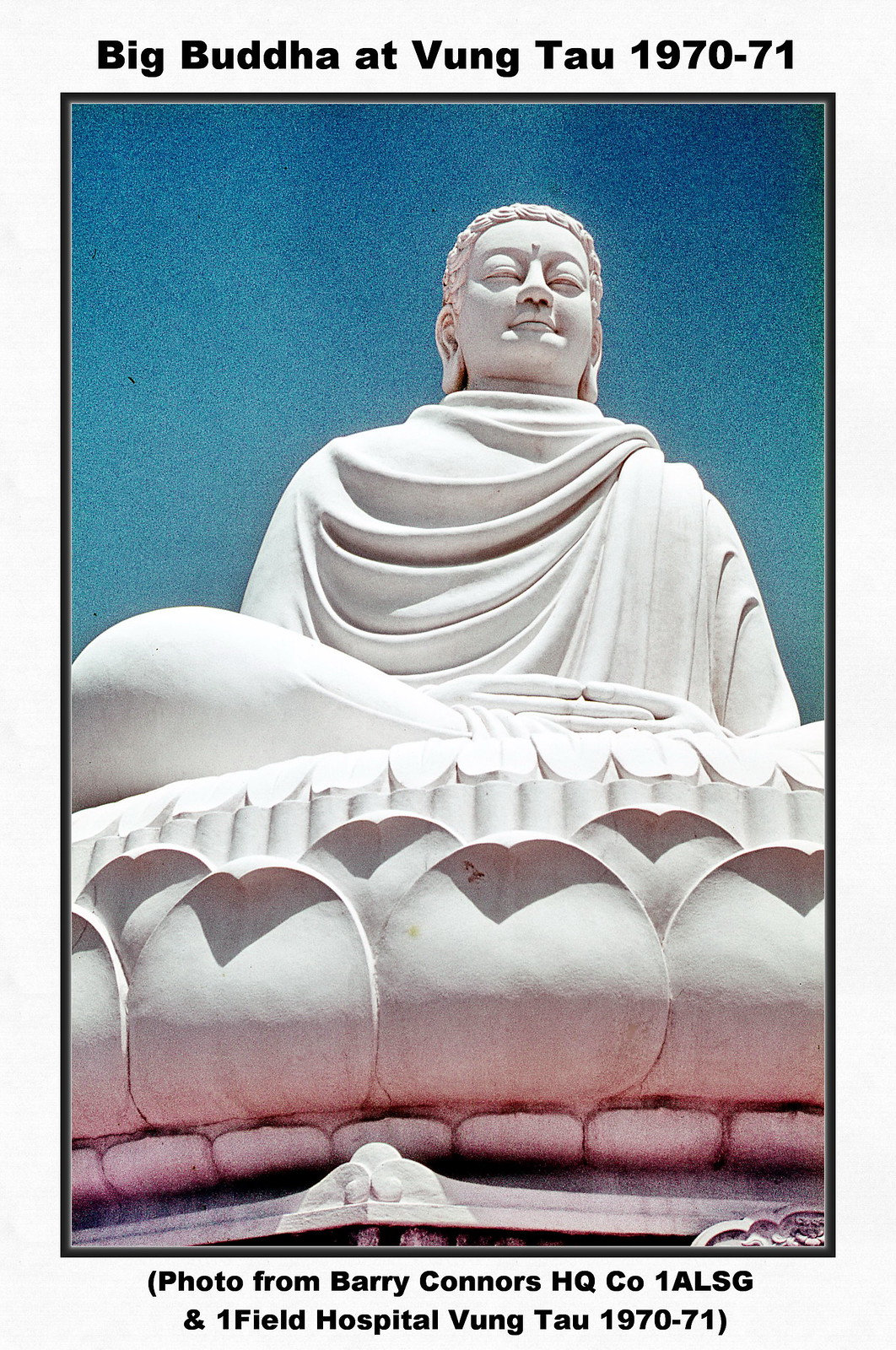This color photograph, taken during the Vietnam War era in 1970-71, captures a serene, large white statue of the Buddha from an upward angle. The title at the top of the photograph reads "Big Buddha at Vung Tau 1970-71," while the bottom of the image is marked with "Photo from Barry Connors HQ, CO 1 ALSG, and One Field Hospital, Vung Tau 1970-71" in parentheses. The Buddha, carved from smooth stone, is seated with crossed legs and folded hands, his eyes peacefully closed, against a brilliant, clear blue sky. The image, framed by a black border, shows leaves overhanging the circular pedestal on which the Buddha rests. The photograph, taken from the base of the statue, emphasizes the enormity and tranquility of the figure.